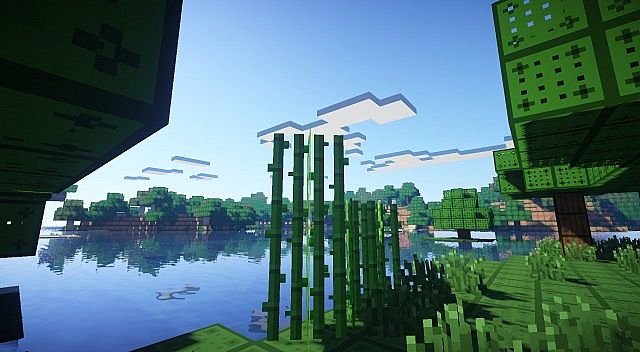In this intricate video game scene, an emerald-hued city emerges, crafted entirely from meticulously arranged green blocks. The city nestles beside a reflective waterfront, with verdant, blocky trees lining the opposite shore, their symmetrical reflections shimmering in the clear water below. A few block-constructed ducks float serenely on the water’s surface, adding life to the pixelated tableau.

In the foreground, tall green posts rise from the ground, accompanied by various other green plants, all sharing the same pixelated block design. Dominating the upper right corner, a large building composed of larger green blocks with cutouts stands prominently, anchored by a brown post at its base.

Beyond the waterfront, majestic block-formed mountains stretch across the horizon, melding into a sky dotted with interconnected square clouds. In the upper left corner, the underside of another cubic building subtly intrudes into the scene, adding depth and complexity to this cleverly crafted virtual world.